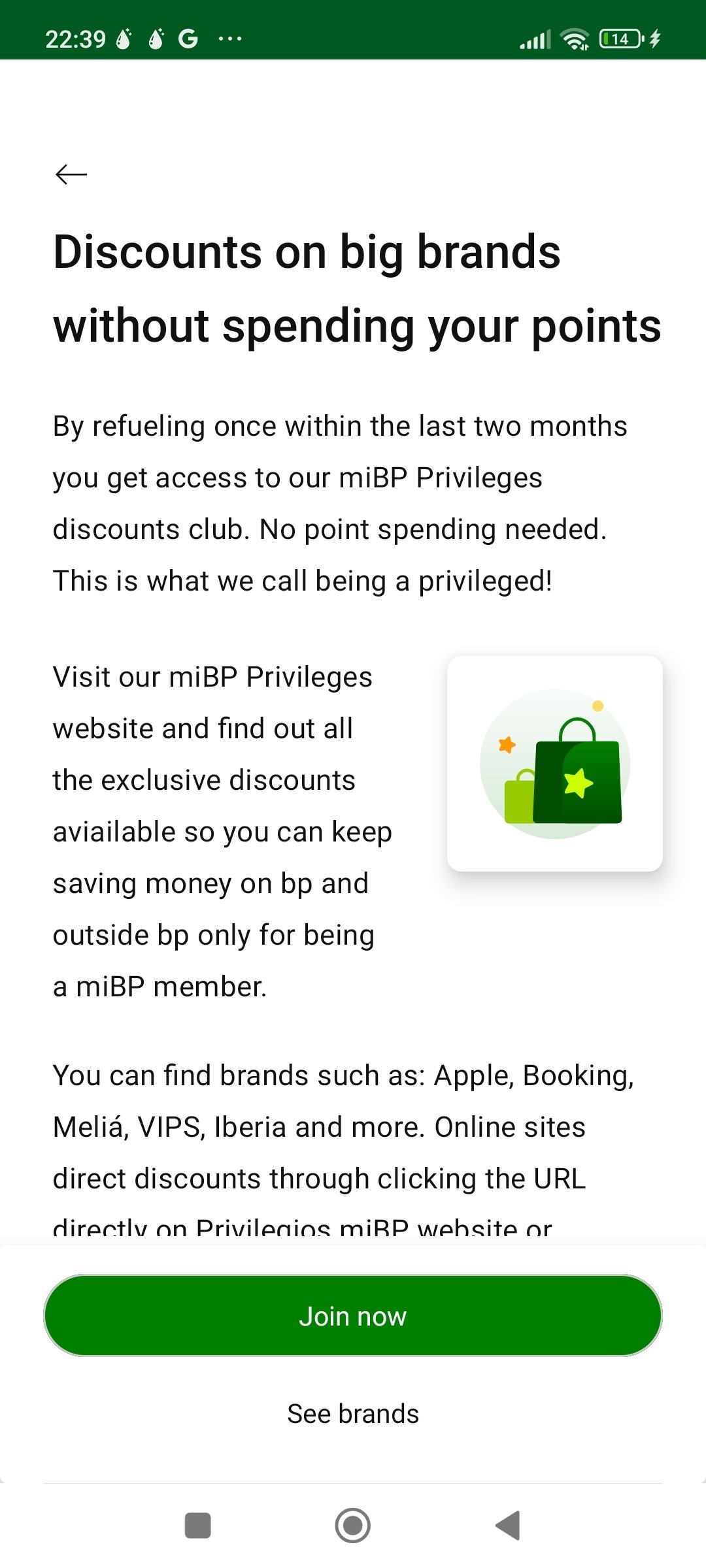This screenshot from a mobile phone illustrates a user interface at 22:39. The top dark green bar includes important status icons. From left to right, it shows the current time, two unidentified icons resembling pairs, a 'G' icon, and an icon with three horizontal white dots. Following these are the Wi-Fi signal icon, mobile signal strength bars, and a battery icon indicating 14% with a thunderbolt, suggesting charging.

Directly below this bar, the screen displays a white page. In the upper left corner, there is a left-pointing arrow. Below the arrow, a message in black font reads: "Discounts on big brands without spending your points. By refueling once within the last two months, you get access to our MIPP Privileges Discount Club. No point spending needed. This is what we call being a privilege."

The message continues to describe the benefits of visiting the MIPP Privileges website, where users will find exclusive discounts on various brands such as Apple, Booking, Melia, Vips, and Iberia. These discounts are available through direct links or online sites, helping MIPP members save money on BP and other brands. Notably, the text contains grammatical errors and unclear phrasing, emphasizing the need for better language crafting.